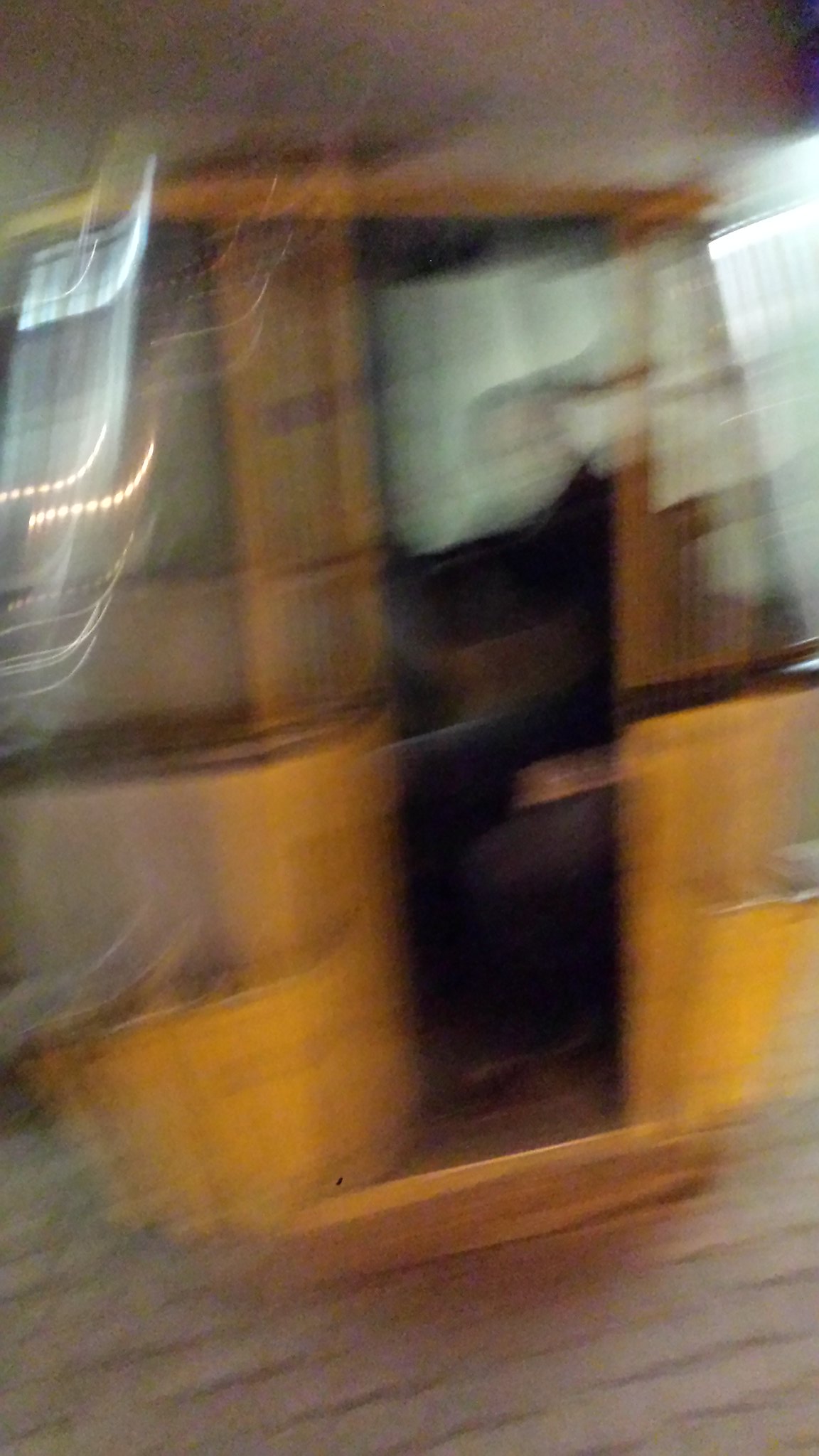In this image, there is a scene with a light-colored wooden floor as the base. At the center is a small yellow structure that resembles a house, equipped with a door. Inside this structure, a black chair is visible, accompanied by various small items scattered around it. The structure appears to be in motion, giving the entire scene a blurred effect, particularly noticeable through the glass around it. The motion has created faint, streaked lines in the image, adding to the sense of speed. In the background, concrete walls stand in contrast to the blurred foreground, suggesting a stationary surrounding environment. A small step leads up into the yellow structure, further emphasizing its resemblance to a tiny house.